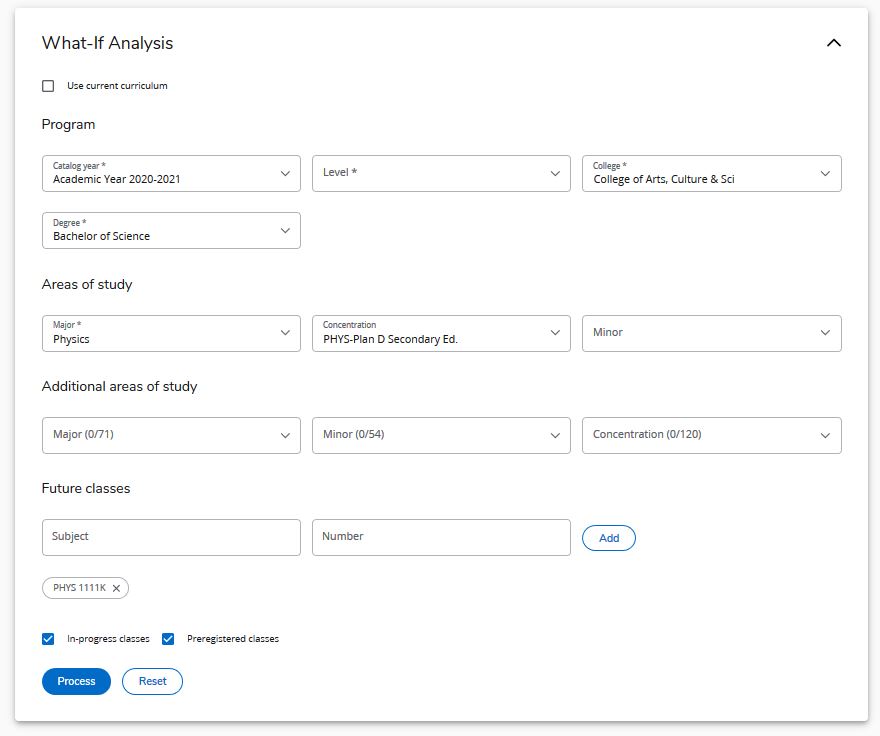The image displays a webpage detailing the planning interface for an academic program. At the top, there's a dropdown menu illustrating the option to collapse or expand the section. The page is focused on "What-If Analysis," advising users to use their current curriculum. This analysis tool is designed to aid in planning one's academic career.

Key sections and selections include:
- **Program:** It allows customization of academic plans, with selected parameters.
- **Current Year/Catalog Year:** Indicates the academic year 2020-2021.
- **Level:** Detailed further by College, specifying the College of Arts, Culture, and Science.
- **Degree:** Bachelor of Science.
- **Major and Concentration:** Physics major with a concentration in Physics Plan D, intended for secondary education teaching.
- **Minor:** No minor selected.
- **Additional Areas of Study:** None beyond the major.

There are specific details about credit completion, hinting at "071, 054, 0 of 120" for the concentration. The interface also includes functionalities for adding future classes, with an example of "Physics 1111K" being added but removable. Options for "In-progress" or "Pre-registered" classes are available, with buttons for "Processed" or "Reset."

In summary, the page provides a comprehensive setup for students to plan and manage their academic courses, ensuring they meet the requirements for their chosen field of study.